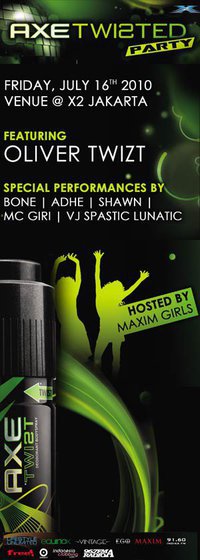The advertisement is a tall, narrow, portrait-oriented poster with a dominant lime green and black background, promoting an event called the "AXE Twisted Party". The word "AXE" is prominently displayed in white letters at the top left, with "TWISTED" in lime green next to it, featuring a distinctive backward "S". Below this, a yellow banner with black lettering announces "PARTY", followed by details in white text: "FRIDAY, JULY 16, 2010," and "VENUE at X2, JAKARTA". There is a section in yellow letters that reads "FEATURING" with "OLIVER TWIST, T-W-I-Z-T" in white, and "SPECIAL PERFORMANCES BY BONE, ADHE, SEAN, MCGIRL, VJ SPASTIC LUNATIC" in white text below.

The bottom section includes the visual elements: a partial image of a tall black AXE Body Spray can to the left, accompanied by silhouettes of two dancing women in yellow, with their arms raised. To their right, a banner reads "Hosted by Maxim Girls" in lime green, against the nightclub-themed background. The overall design combines photographic product elements and colorful graphic illustrations, creating an energetic and vibrant promotional piece.